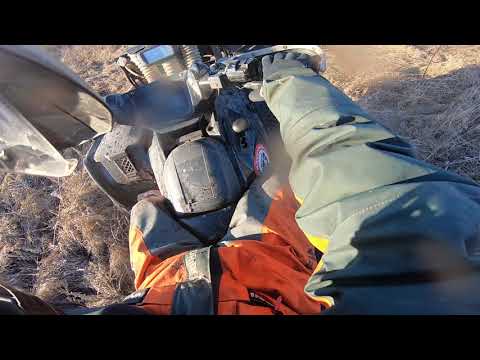The image captures a dynamic scene taken from the perspective of a person riding an ATV, likely using a GoPro mounted next to their visor. The rider is wearing an orange reflective jumpsuit with gray pants made of a heavy, possibly rubber or vinyl material. Their left hand, clad in a heavy-duty glove, is visible outstretched towards the handlebars, while their right hand grips one of the gears, as the vehicle appears to be in motion. The ATV itself looks old and dirty, suggesting it has been driven through muddy terrain. In the background, the landscape consists of dry, beige grass, which implies a dry season or winter setting. The console of the ATV is gray and includes a screen or interface, possibly resembling a phone, providing additional functionality. The overall scene depicts an adventurous off-road experience, highlighted by the rider’s rugged appearance and the challenging environment.